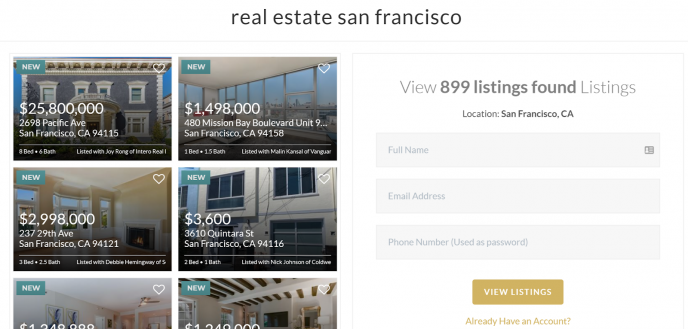This image showcases a real estate advertisement displayed against a crisp white background, prominently featuring the San Francisco housing market. A delicate blue line horizontally divides the image, above which six thumbnails of various San Francisco houses are arranged. These include properties listed at $25,800,000, $1,498,000, $2,298,000, and $3,600,000, alongside two partially visible listings at the bottom. Each property thumbnail is adorned with a blue "New" label and a small white heart icon.

On the right side of the image, text indicates the availability of "899 listings found" in San Francisco, California, accompanied by a section for customer interaction. This section includes input fields for the user's name, email address, and phone number, with a prominent brown "View Listings" button inviting further exploration.